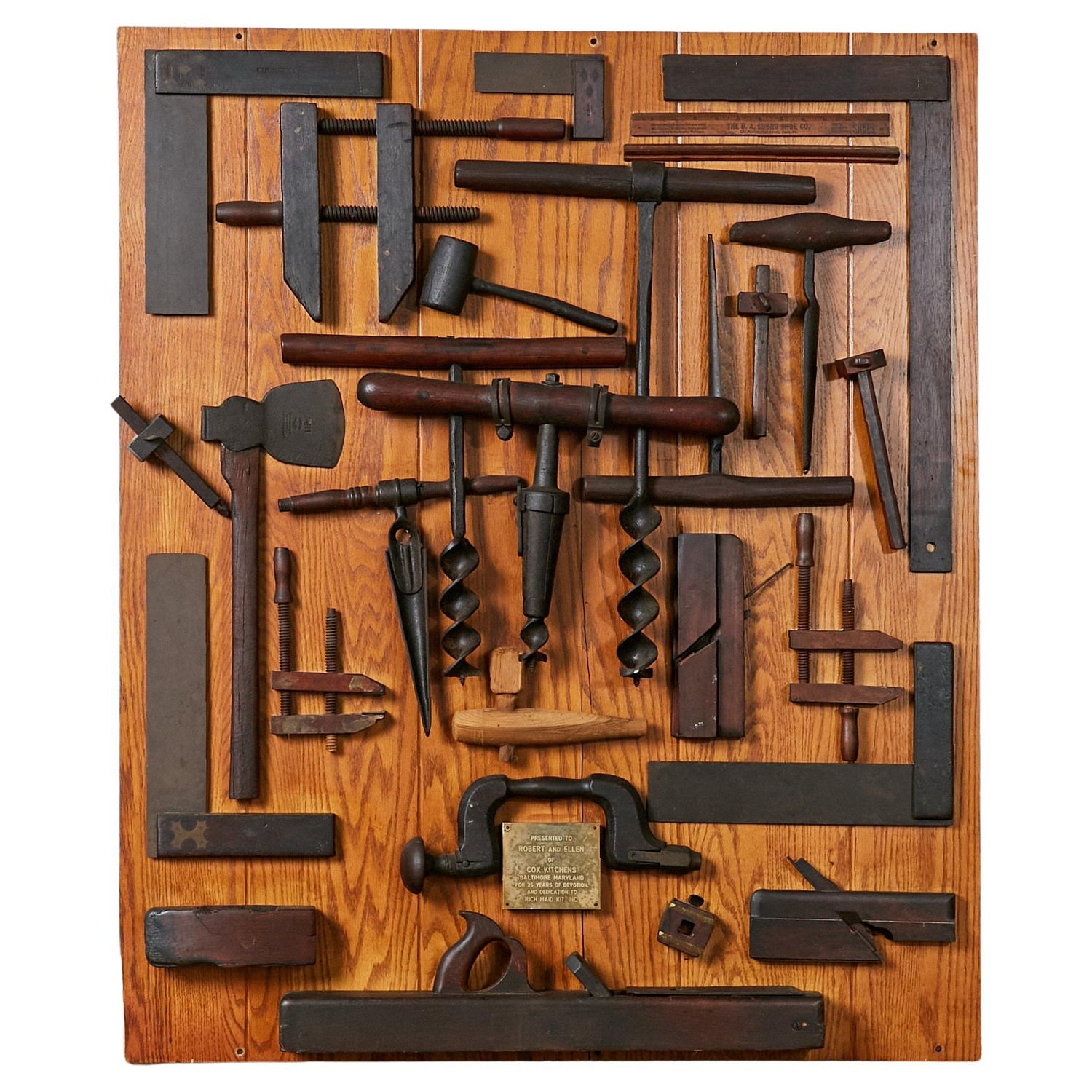This indoor photographic image captures a meticulous display of vintage hand tools arranged neatly on a weathered brown wooden wall. Prominently featured are an array of levels in the top corners, flanked by L squares on each side. Centrally placed between the L squares, several wood clamps and brace drills with two handles are visible. Additionally, the collection includes multiple hammers, hand drills, a plane, and an axe. The tools, predominantly dark black iron with some wooden handles, exude an aged quality and serve a variety of woodworking functions. At the bottom of the display is a small plaque that reads, "Presented to Robert and Ellen of Cox Kitchens, Baltimore, Maryland," though finer text is too small to decipher. The overall scene evokes a sense of historical craftsmanship, emphasizing both the functional and aesthetic aspects of these old woodworking tools.